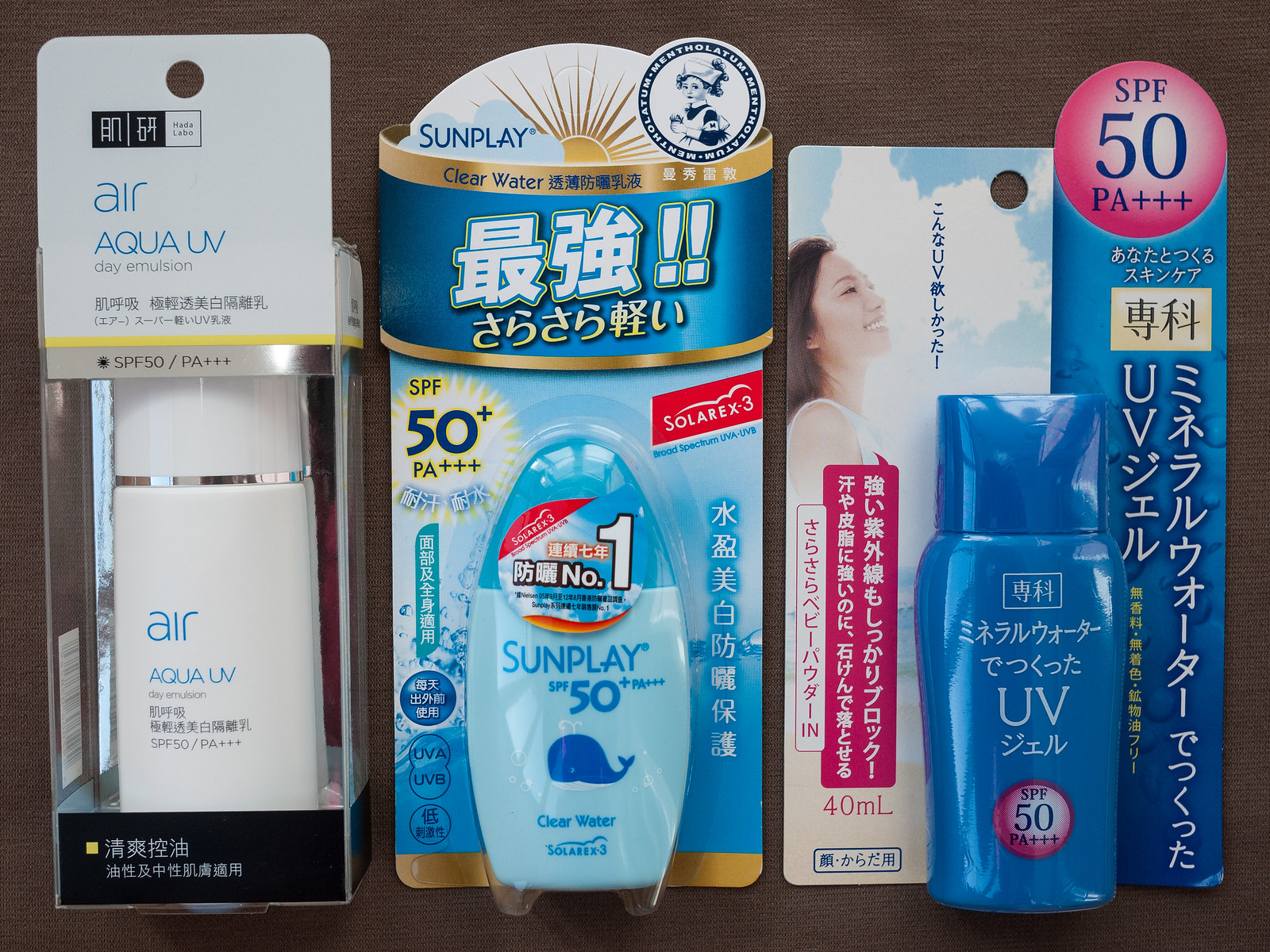In this detailed image, there are three distinct products, likely of Chinese or Japanese origin, displayed against a smooth, brownish background, possibly a table surface or bed sheet. Each product is encased in its own packaging, and they are arranged from left to right.

On the left, the first product features a predominantly white packaging. It consists of a clear, plastic box housing a white, rectangular tube with a silver-banded lid. The tube prominently displays the word "air" in lowercase blue letters, followed by "Aqua UV" in uppercase blue letters. Below this, there's black text with Chinese characters and the marking "SPF 50/PA+++." The top of the box has a black and white logo with the text "AN54" in white, and repeats the product name in the same blue and black font arrangement: "air," "Aqua," and "Day Emulsion." Additional Chinese script appears at the bottom, surrounded by a black border with yellow and white text.

The central product is packaged in a blue cardboard backing, displaying a small sunscreen bottle affixed to the front. The bottle itself is two-toned with a darker blue rounded cap and a lighter blue body. It is labeled "Sunplay SPF 50+ PA+++" in darker blue text, accompanied by an image of a blue whale. Underneath this image, the words "clear water" are visible. The packaging includes further writing in Chinese or Japanese, with key details like "SPF 50+ PA+++" highlighted in blue with a yellow outline. The product name is written in white Chinese characters over a blue ribbon.

On the right, the final product is contained in a tall, rectangular, blue cardboard box, presenting another sunscreen bottle. This bottle is a deeper blue and taller in shape, featuring "UV" in white letters on its front, surrounded by more Chinese or Japanese characters. A prominent pink circle on the bottle signifies "SPF 50 PA+++" in black text. The sides of the box show vertical lines of additional writing in Chinese or Japanese, while a second pink circle at the upper right corner of the packaging reiterates "SPF 50 PA+++" in dark blue.

The meticulous layout and vibrant packaging designs collectively communicate a clear message about sun protection, emphasizing the products’ efficacy and cultural origins.